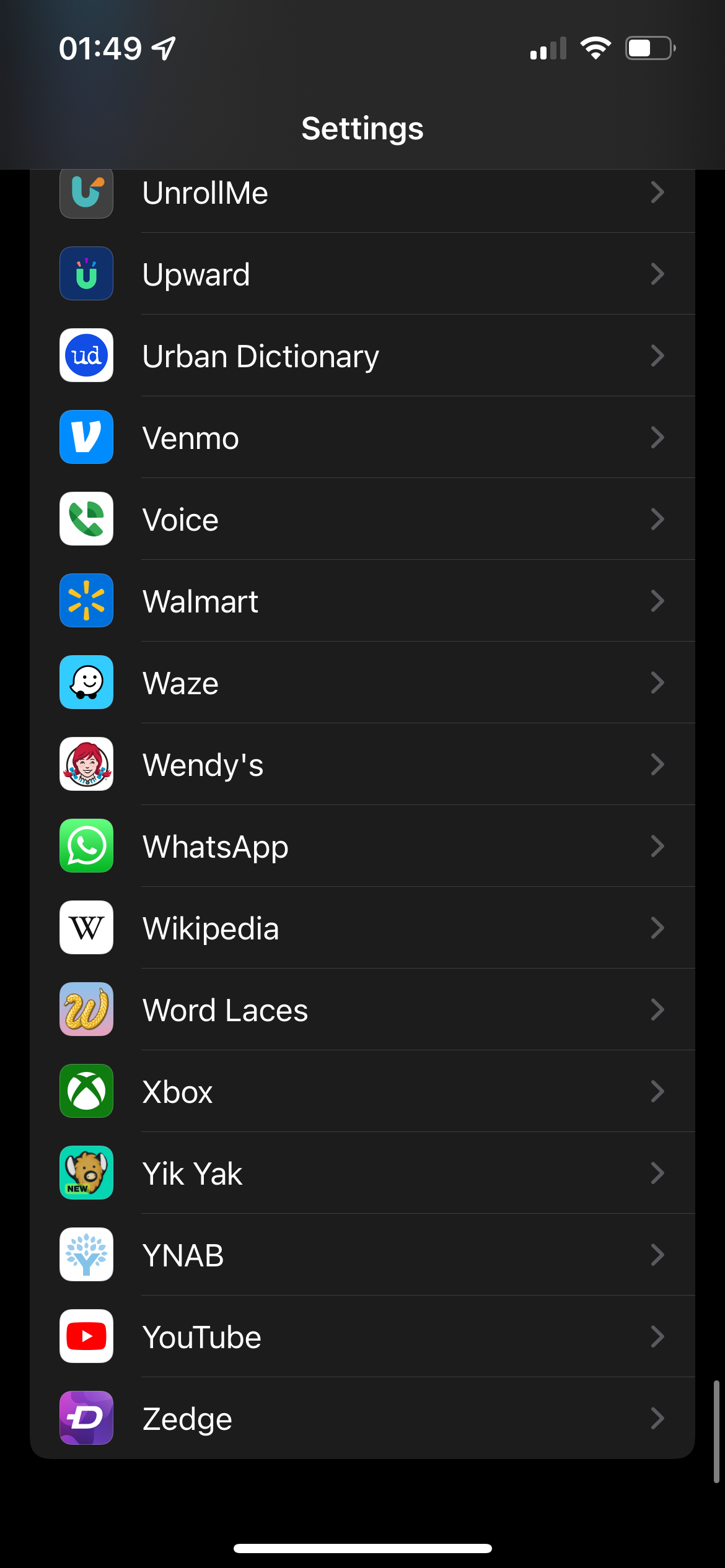Screenshot of an iPhone’s Settings Page

The screenshot displays an iPhone's settings interface. The status bar at the top of the screen shows the time as 1:49 in the upper left corner, accompanied by a small leftward arrow. On the upper right side, it indicates strong cellular signal bars, full Wi-Fi signal, and a battery icon showing approximately 50% charge. The entire background is black, with white text for high contrast.

Below the status bar, the header "Settings" is prominently featured. Beneath this, a list of applications is visible, each accompanied by its respective icon on the left and a clickable rightward arrow on the right. The applications listed include:

- Unroll.me
- Upward
- Urban Dictionary
- Venmo
- Voice
- Walmart
- Waze
- Wendy's
- WhatsApp
- Wikipedia
- Word Laces
- Xbox
- Yik Yak
- YNAB (You Need a Budget)
- YouTube
- Zedge

Finally, at the bottom of the screen, there's a small white horizontal line, suggesting the option to swipe up and close the current window.